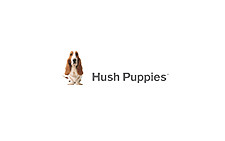The image depicts a small logo for the Hush Puppies brand, featuring a front-facing Basset Hound with distinct characteristics. The dog has long, brown ears, a white face with a black nose, and black eyes. Its body is primarily white with subtle brown markings. To the right of the dog, the text "Hush Puppies" is displayed in black font, starting with a capital 'H' and 'P.' The entire logo is set against a plain white background, with no additional elements, giving it a simple and clear appearance.